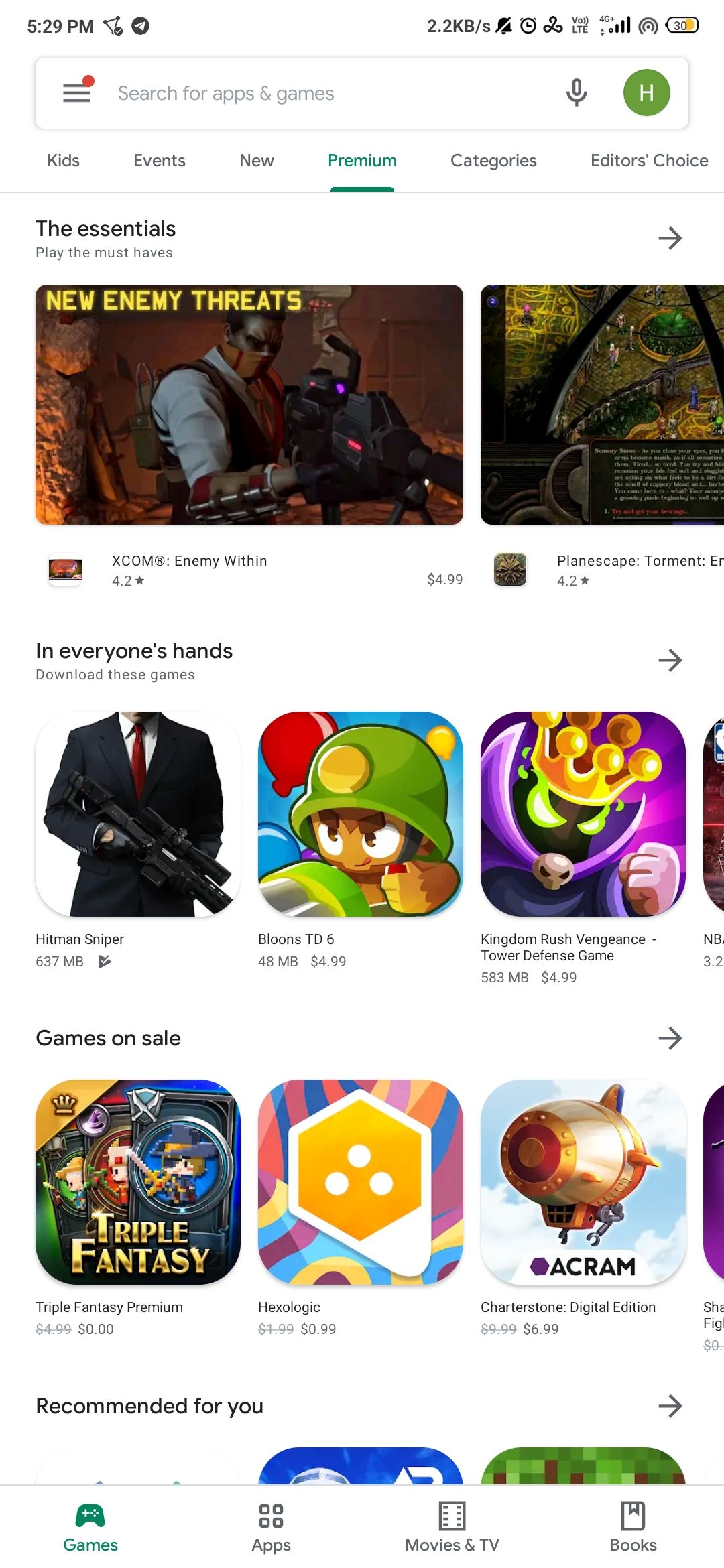The image depicts a smartphone screen showcasing a digital storefront, specifically highlighting the 'Premium' section for apps and games. At the top of the screen, the time is displayed as 5:29, along with various status indicators including battery percentage and data usage (2.2 kb). Below these indicators, there's a search bar labeled "Search for apps and games," accompanied by a gray microphone icon and an icon resembling an 'eight' on a green background.

The screen features several navigation categories including Kids, Events, New, Premium, Categories, and Editor's Choice, with 'Premium' being the currently active section. Within this section, a headline reads "The Essentials, play the must-haves," showcasing notable apps and games.

The first featured app is "XCOM: Enemy Within," displaying a character holding a large weapon, giving off a superhero or villain vibe. Another highlighted app is "Planescape: Torment," which boasts a 4.2-star rating and appears to be a text-based game. Additional app icons presented include "Hitman Sniper," "Bloons TD6," "Kingdom Rush Vengeance," and "Triple Fantasy Premium."

Towards the bottom of the screen, navigational icons for Games, Apps, Movies & TV, and Books are visible. The background of the image is predominantly white, contrasted by an array of colorful app icons, primarily depicting various games.